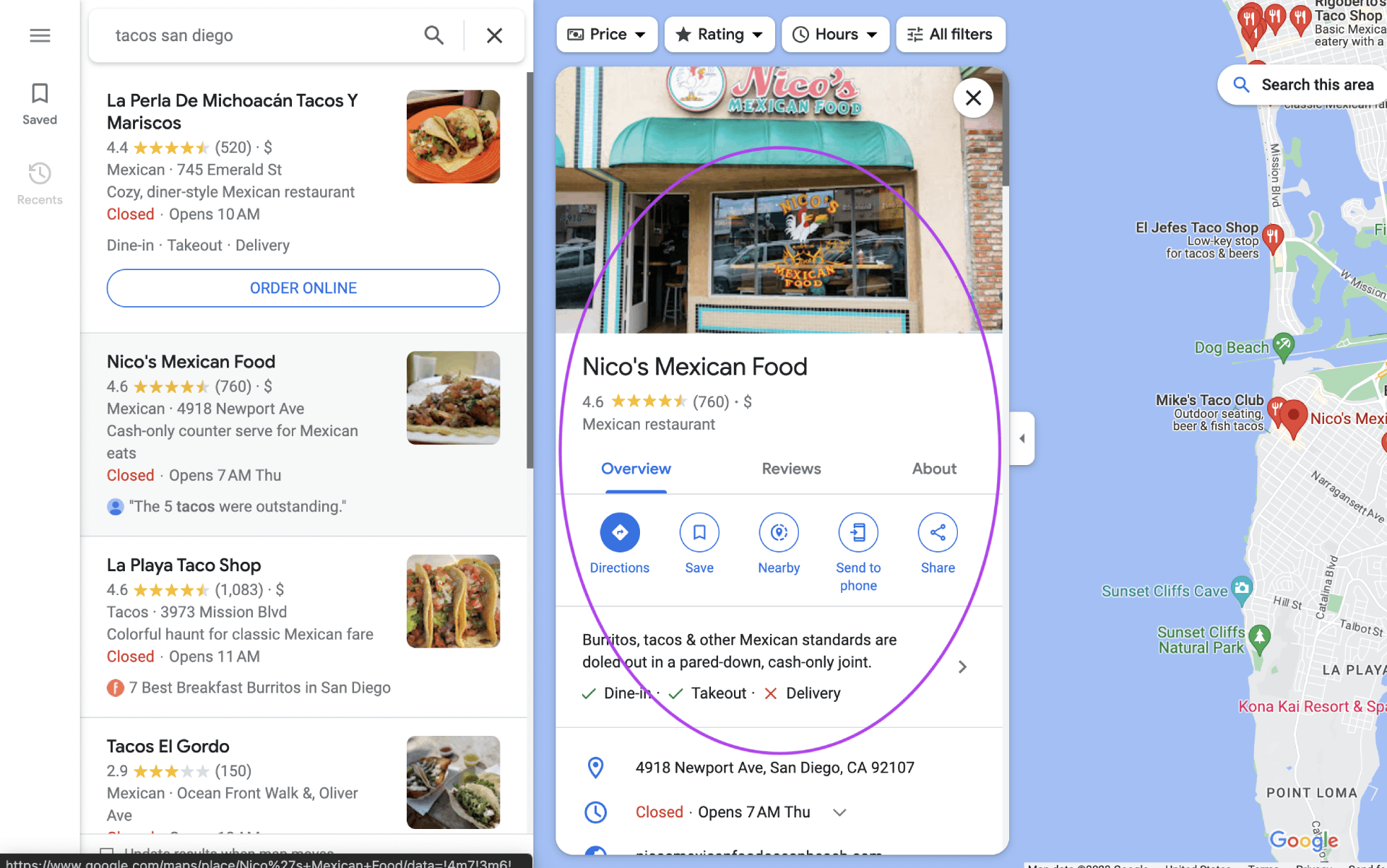The image is a screenshot from Google Maps showcasing several taco restaurants in San Diego. On the left side of the image, there is a menu tab with three horizontal lines, followed by "Saved" and "Recents" options, each with corresponding icons. Below is a search bar displaying "Tacos San Diego."

The search results highlight four distinct taco spots:

1. **La Perla Taco & Mariscos**
   - **Rating:** 4.4 stars, 520 reviews
   - **Price Range:** $
   - **Type:** Mexican
   - **Address:** 745 Emerald Street
   - **Description:** Cozy, diner-style Mexican restaurant
   - **Status:** Closed, opens at 10 a.m.
   - **Services:** Drive-in, Takeout, Delivery
   - **Image:** Features a photograph of tacos
   - **Option:** "Order Online"

2. **Mico's Mexican Food** (Highlighted)
   - **Rating:** 4.6 stars, 760 reviews
   - **Price Range:** $
   - **Type:** Mexican
   - **Address:** 4918 Newport Ave
   - **Description:** Cash-only, counter-serve Mexican eatery
   - **Status:** Closed, opens at 7 a.m. on Thursday
   - **Review Highlight:** "The five tacos were outstanding"
   - **Image:** Close-up photo of tacos

3. **La Playa Taco Shop**
   - **Rating:** 4.6 stars, 1,083 reviews
   - **Price Range:** $
   - **Type:** Tacos
   - **Address:** 3973 Mission Blvd
   - **Description:** Colorful spot known for classic Mexican fare
   - **Status:** Closed, opens at 11 a.m.
   - **Highlight:** "Seven best breakfast burritos in San Diego"
   - **Image:** Close-up photo of tacos

4. **Tacos El Gordo**
   - **Rating:** 2.9 stars, 150 reviews
   - **Type:** Mexican
   - **Address:** Ocean Front Walk and Oliver Ave
   - **Image:** Photo of tacos

The main section at the top features Mico's Mexican Food in detail:

- **Image:** Storefront of Mico's
- **Restaurant Information:** Repeated details from the search result
- **Tabs:** Overview, Reviews, About
- **Buttons:** Directions, Save, Nearby, Center, Phone, Share
- **Description:** "Burritos, tacos, and other Mexican standards are doled out in a pared-down, cash-only joint."
- **Status:** Closed, opens at 7 a.m.
- **Services:** Dine-in (green arrow), Takeout (green arrow)
- **Address:** 4918 Newport Ave, San Diego, CA 92107
- **Map:** Displayed on the right, showing the geographical area

Overall, the screenshot comprehensively displays various taco restaurants with ratings, reviews, operational status, and images of tacos, offering an organized look at options in San Diego.